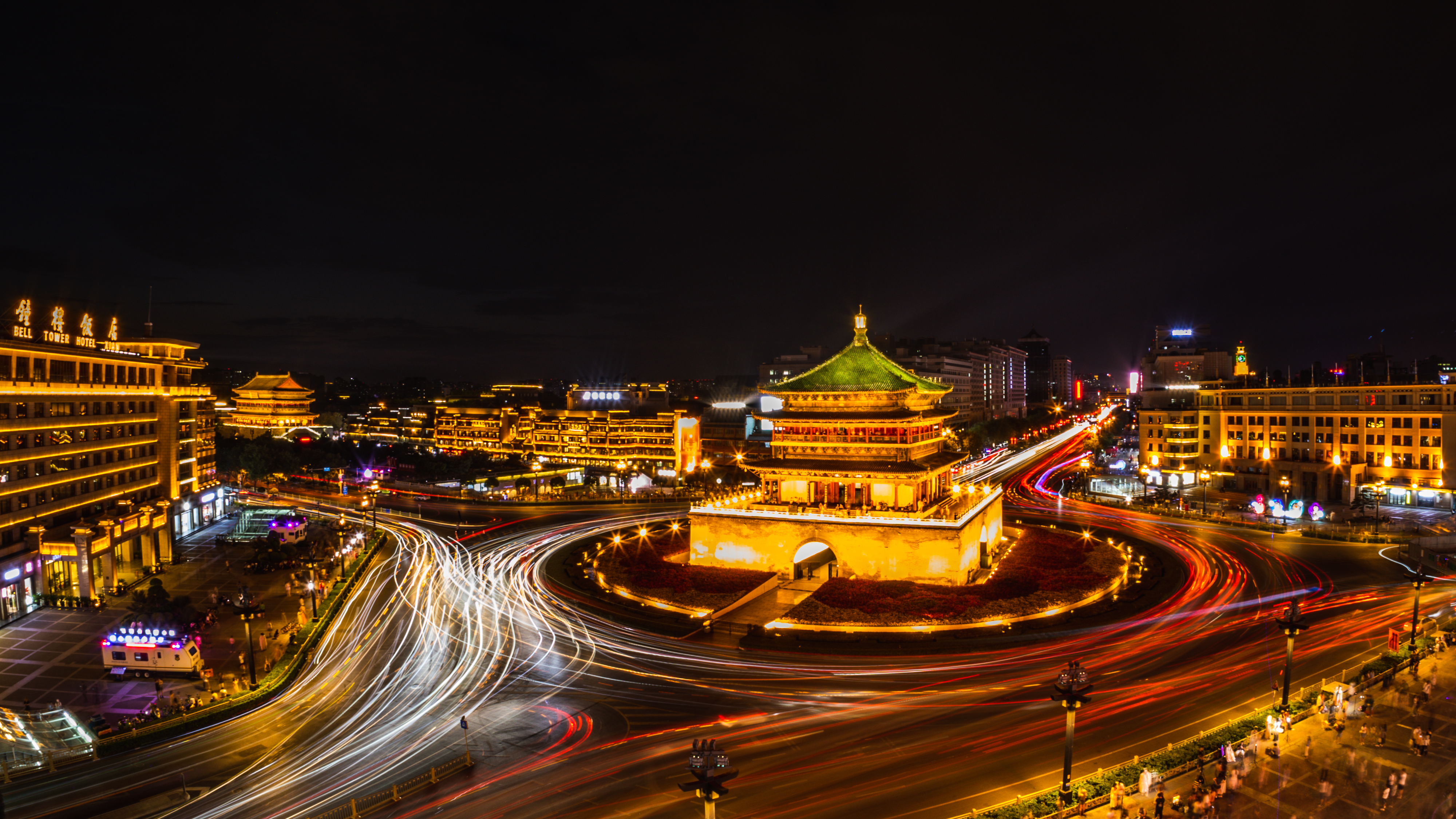This vibrant nighttime time-lapse photograph captures the bustling essence of an Asian city, characterized by distinctive Chinese architecture and illuminated signage in Chinese characters. At the heart of the image lies a prominent, circular Chinese-style temple with a green roof, set within a busy roundabout. The long exposure technique transforms the car lights on the roadways into dynamic white and red streaks, resembling a flowing river of light. Surrounding the temple, a mix of lit buildings adds to the lively city atmosphere, including what seems to be hotels and other structures, though the skyline remains relatively low without any skyscrapers. In the bottom right, a walkway with lampposts and greenery is populated with people, suggesting a popular tourist or gathering area. The overall scene conveys a vibrant city, perhaps a tourist-friendly destination brimming with cultural sites and bustling activity.